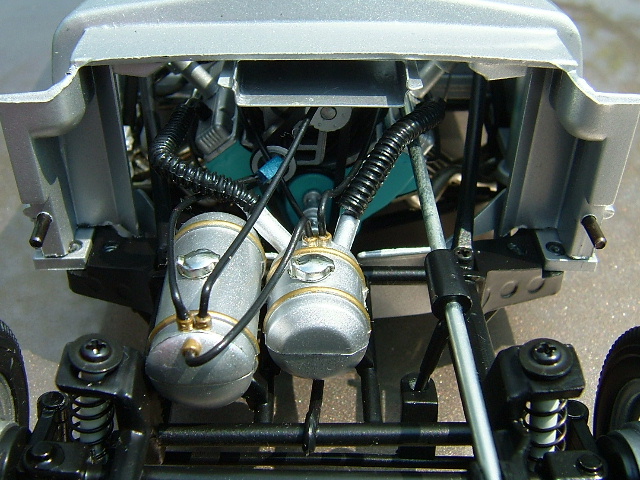In this detailed image, we see the intricate setup of an automotive engine bay with a focus on its electronic and mechanical components. At the center, there are two prominent silver cylindrical containers. The one on the left is slightly larger and more chrome-colored, featuring a silver cap with speckles and accented by gold rings at both its front and back ends. This larger container has three black tubes extending from it towards the front of the vehicle. The smaller, right-side container also boasts a chrome cap and gold rings, but appears a bit fatter and has two black pipes attached, which connect to bendable black tubes leading to the vehicle's front.

Both containers are firmly integrated into the main engine structure, supported by visible black coils and wires. Surrounding these components, on either side of the picture, are black screws securing silver handles that are part of a rounded rectangular compartment housing the electrical elements. This compartment includes several wires and coiled wires, some resembling transistor or resistor parts. Lower down in the image, the vehicle's gray casing is visible alongside the bottom corners where the tires and suspension components, including black-painted springs and shock absorbers, are viewable. A connecting metal rod runs between the tires, providing critical support. Each spring casing has a bolt designed for a hexagon screwdriver, highlighting the detailed engineering and assembly of this machinery.